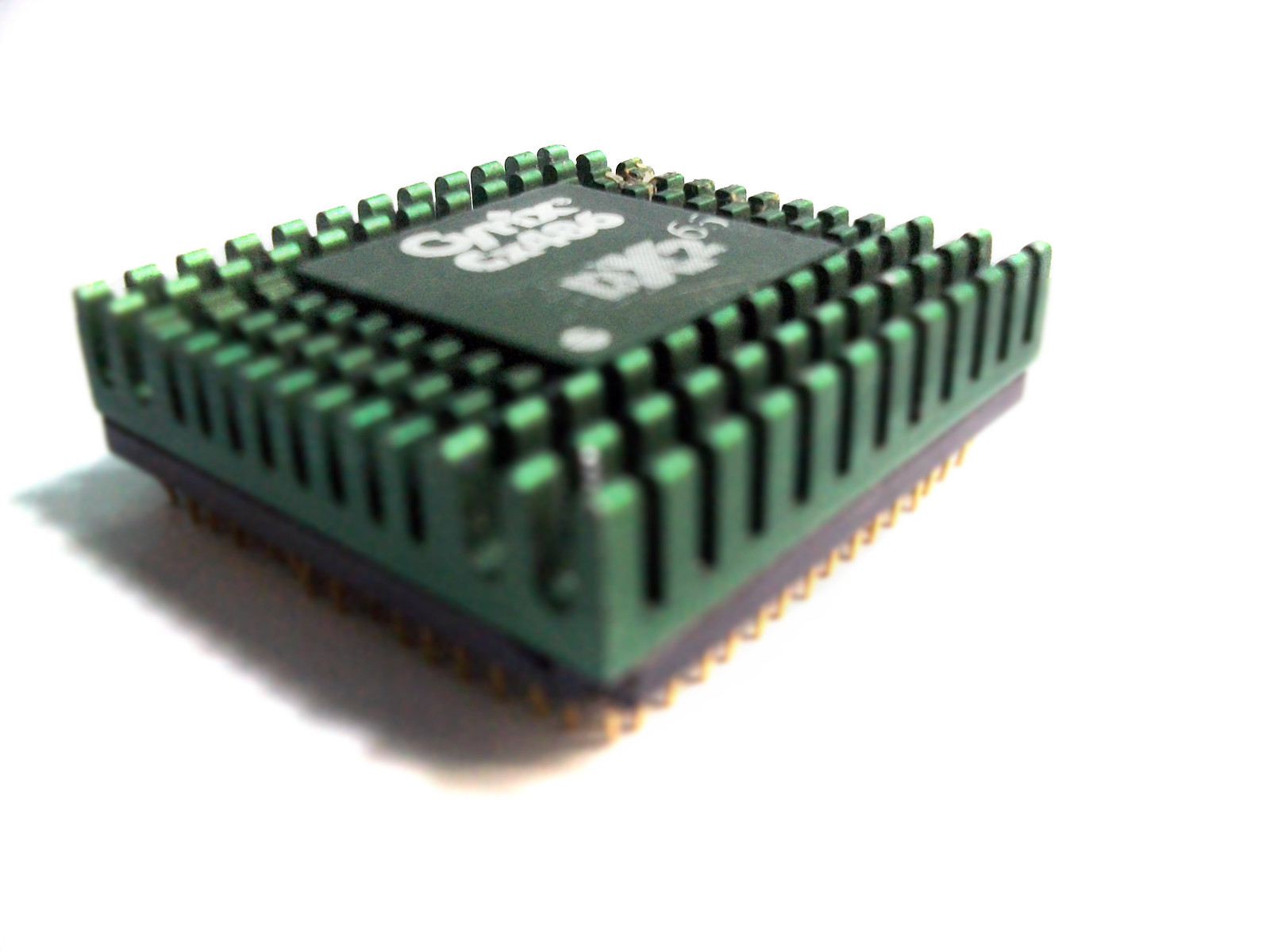The photograph showcases a close-up of a multi-layered microchip set against a plain white background. The microchip comprises three distinct levels: the base is yellow, featuring short yellow wires peeking out at the bottom, followed by a flat purple platform in the middle. The topmost layer is a green square component adorned with intricate indentations and protrusions. At the very top, a smaller dark green square is fixed, displaying the barely legible text "DX26." The overall construction casts a noticeable shadow to the left on the white surface, accentuating the microchip's layered complexity. The image appears somewhat blurry, especially when viewing the intricate details of the computer chip.